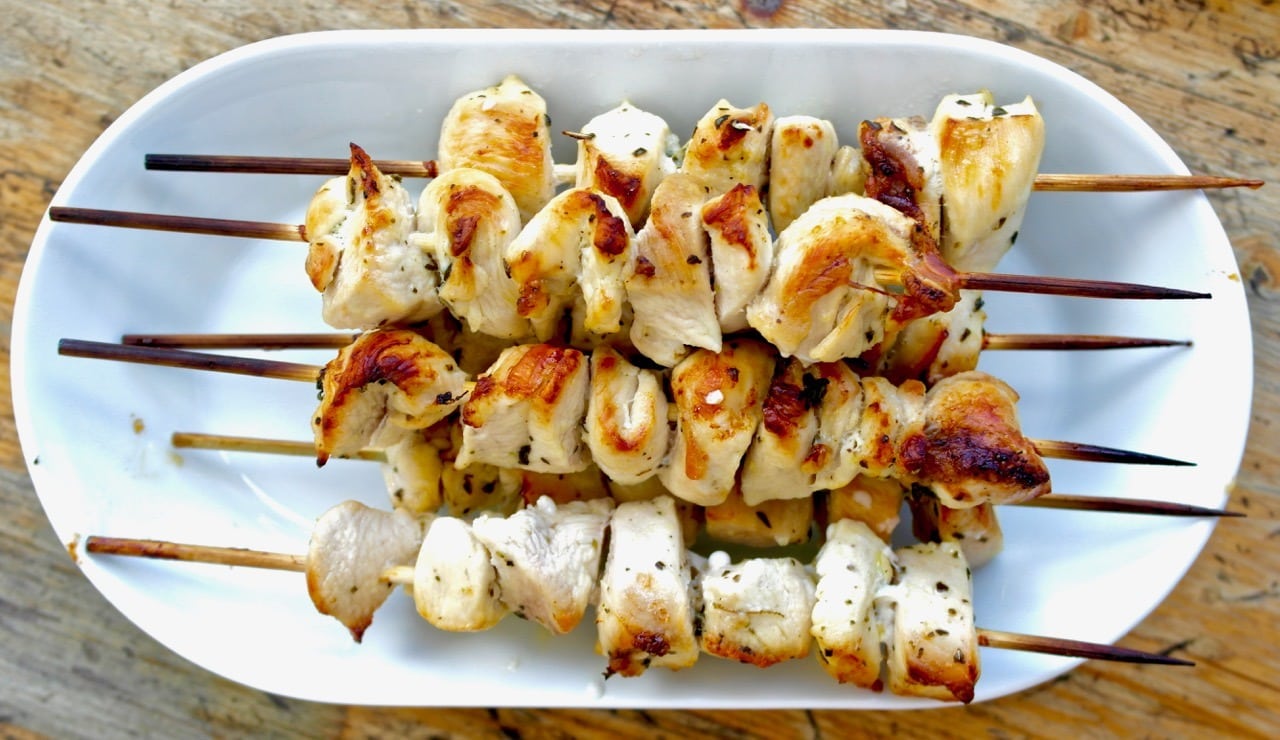The image showcases six shish kebabs neatly arranged on a white, rounded rectangular plate placed on a brown wooden table. The skewers, each charred at the edges and of varying lengths, feature cooked chicken pieces that are browned, with some displaying charred black spots, indicating grilling. The sticks, themselves bearing brown burn marks, support the meat, which visibly alternates between well-cooked brown parts and lighter, less cooked sections. A faint sauce stain can be seen on the left side of the plate, adding an element of rustic dining to the presentation. The composition is horizontally aligned, with the skewers positioned at different angles, creating a dynamic yet orderly presentation.